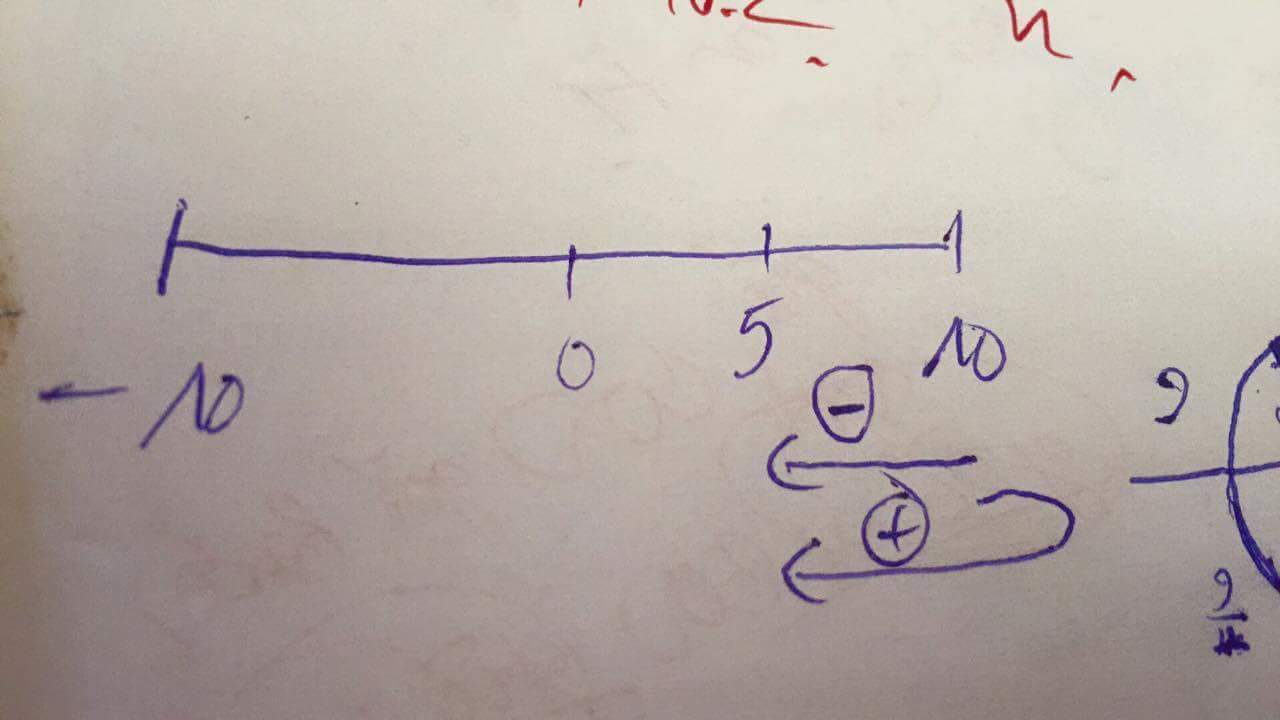This is a color photograph showcasing a piece of white paper with various mathematical notations and markings in blue and red ink. Dominating the image is a horizontal blue ink line marked with four key points: from left to right, the points are labeled "No" or "No. above zero", "0", "5", and an ambiguous "above zero". Adjacent to the leftmost point is a line resembling a negative sign, potentially indicating a negative value above zero. Beneath this main scale, there are additional markings including a distinct negative sign and a positive sign, each associated with two lines. The paper also features other miscellaneous mathematical writing in blue ink.

Additionally, there are some illegible red ink squiggles positioned above the scale on the left side, further adding to the complexity of the image. On the right side of the paper, there are faint writings, barely discernible, contributing to the overall sense of mathematical exploration. No coherent words are visible, leaving the focus purely on the numerical and symbolic notations scattered across the paper.